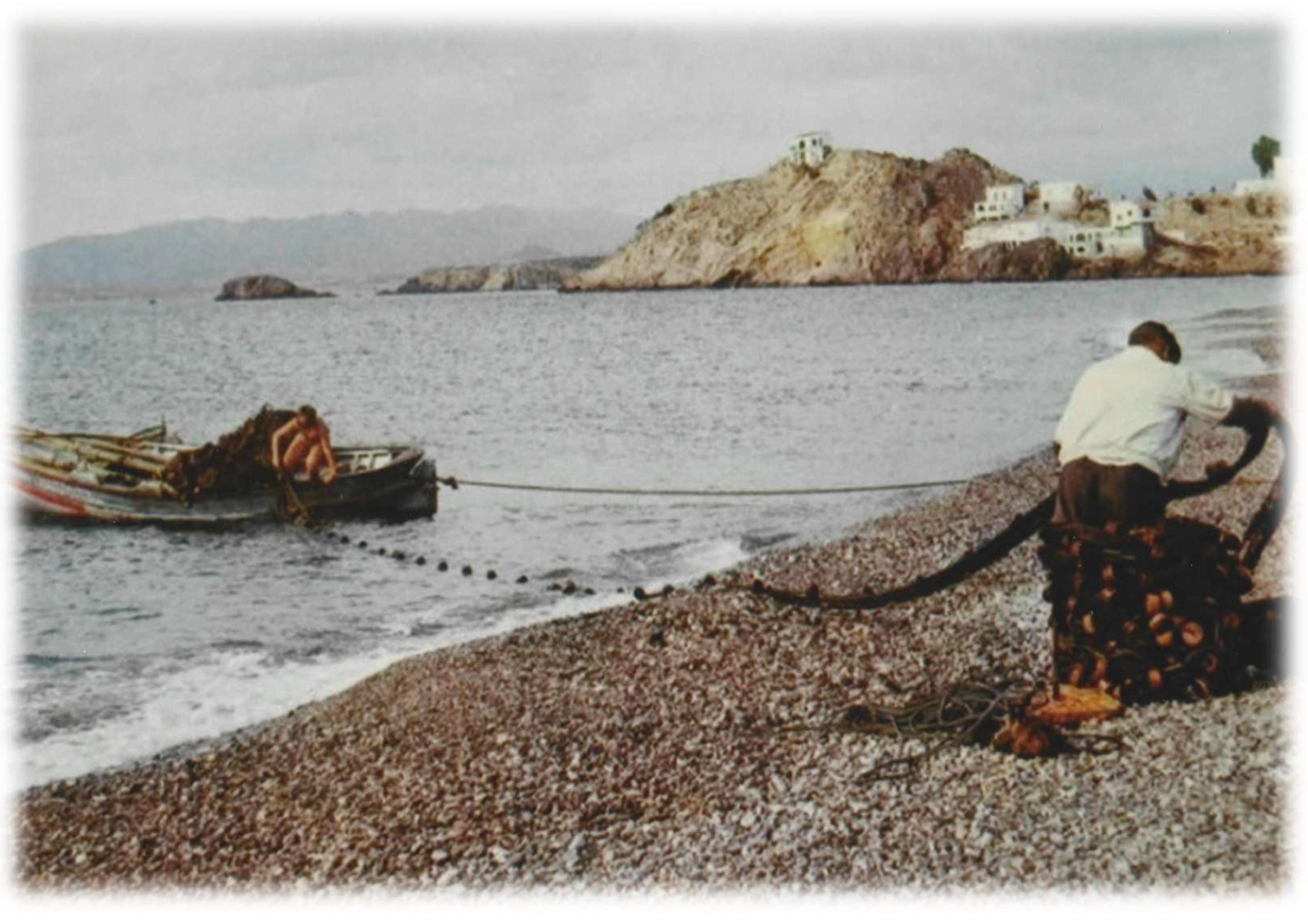This horizontally aligned rectangular digital image, which appears to be a screenshot of a painting, depicts a coastal scene with grainy edges. The foreground features a shoreline composed of numerous small, gravel-like rocks, occupying the lower right-hand corner and spreading across the bottom. A man, wearing a white shirt and dark pants, stands on the rocks, handling a rope or fishing net that wraps around the lower part of his legs. The other end of the rope or net extends into the water, where it is held by a person in a small, canoe-shaped boat in the shallow area. The person in the boat appears to be wearing minimal clothing, possibly a bikini, and is attending to multiple buoys interspersed across the rope. The boat is white with a red stripe. In the background, gray clouds cover the sky above a hilly area that stretches from the middle to the far right of the image. The hillside is dotted with a couple of houses and some green patches, suggesting trees or vegetation. The primary colors of the image are brown, gray, blue, black, and touches of green, lending an overall muted and possibly antiquated appearance.